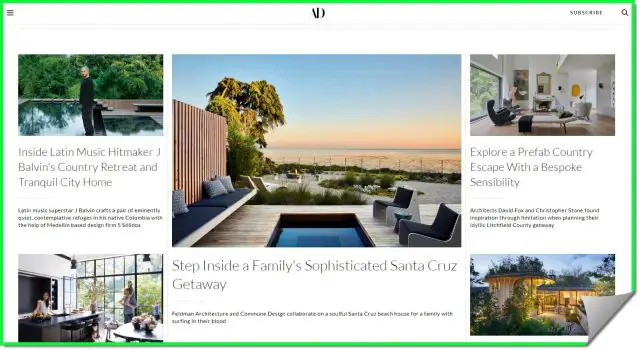This image showcases a stylishly designed website with a green border encasing the page and a distinctive folded corner in the bottom right. At the top, the site features "A" and "D" in black font, with a "Subscribe" button in the upper right corner and a three-line (hamburger) menu icon in the upper left.

The main content area displays a series of high-quality images and their corresponding descriptions. The first image features a man dressed in black, standing in front of a pool, accompanied by the text: "Inside Latin music's hit maker J Balvin's Country Retreat and Tranquil City Home." 

The second image depicts an outdoor patio seating arrangement overlooking a beach framed by tropical trees, under a pinkish sunset. The caption reads: "Step inside a family's sophisticated Santa Cruz getaway."

In the upper right of this section is a photo of a modern home with white and black furniture and an oak wood floor. Its caption states: "Explore a prefab country escape with a bespoke sensibility."

Additional images include a bar area with a sleek black countertop and a couple of people visible inside a room featuring large glass windows that reveal lush greenery outside.